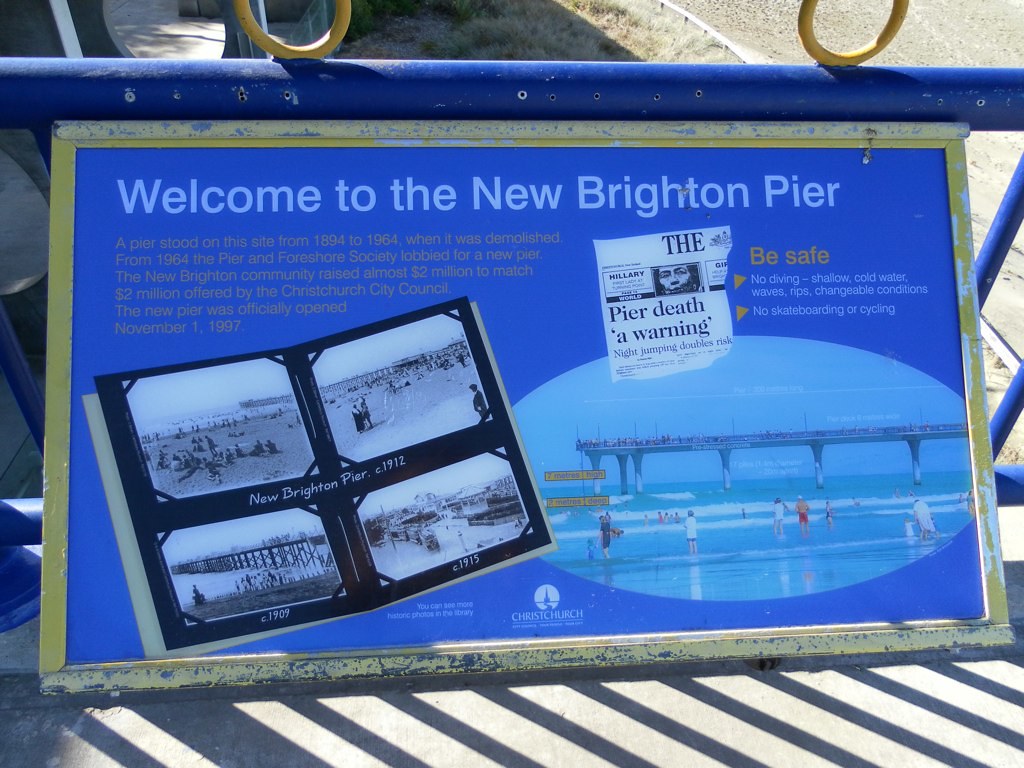The image depicts a detailed, landscape-oriented color photograph of a welcome sign for the New Brighton Pier, prominently mounted on a blue and yellow metal railing. The sign's typography at the top announces, "Welcome to the New Brighton Pier" in white letters on a blue background. Below this greeting, on the left, there is small, difficult-to-read text followed by an open photo album-like illustration showcasing four black and white vintage photographs of the pier from the years 1909, 1911, 1912, and 1915. Centered above these photos is the label "New Brighton Pier, circa 1911." To the right of the photo album, an oval illustration displays a modern, colored photograph of the pier with contemporary swimmers in white clothing and shorts. Adjacent to this, a newspaper clipping headlined "Pier Death: A Warning" highlights safety alerts, advising on dangerous conditions such as no diving, shallow and cold water, waves, rips, and changeable conditions, along with prohibitions against skateboarding and cycling. The sign's weathered frame, originally blue and yellow to match the railing, carries a mix of shadows from the metal bars due to sunlight filtering through.